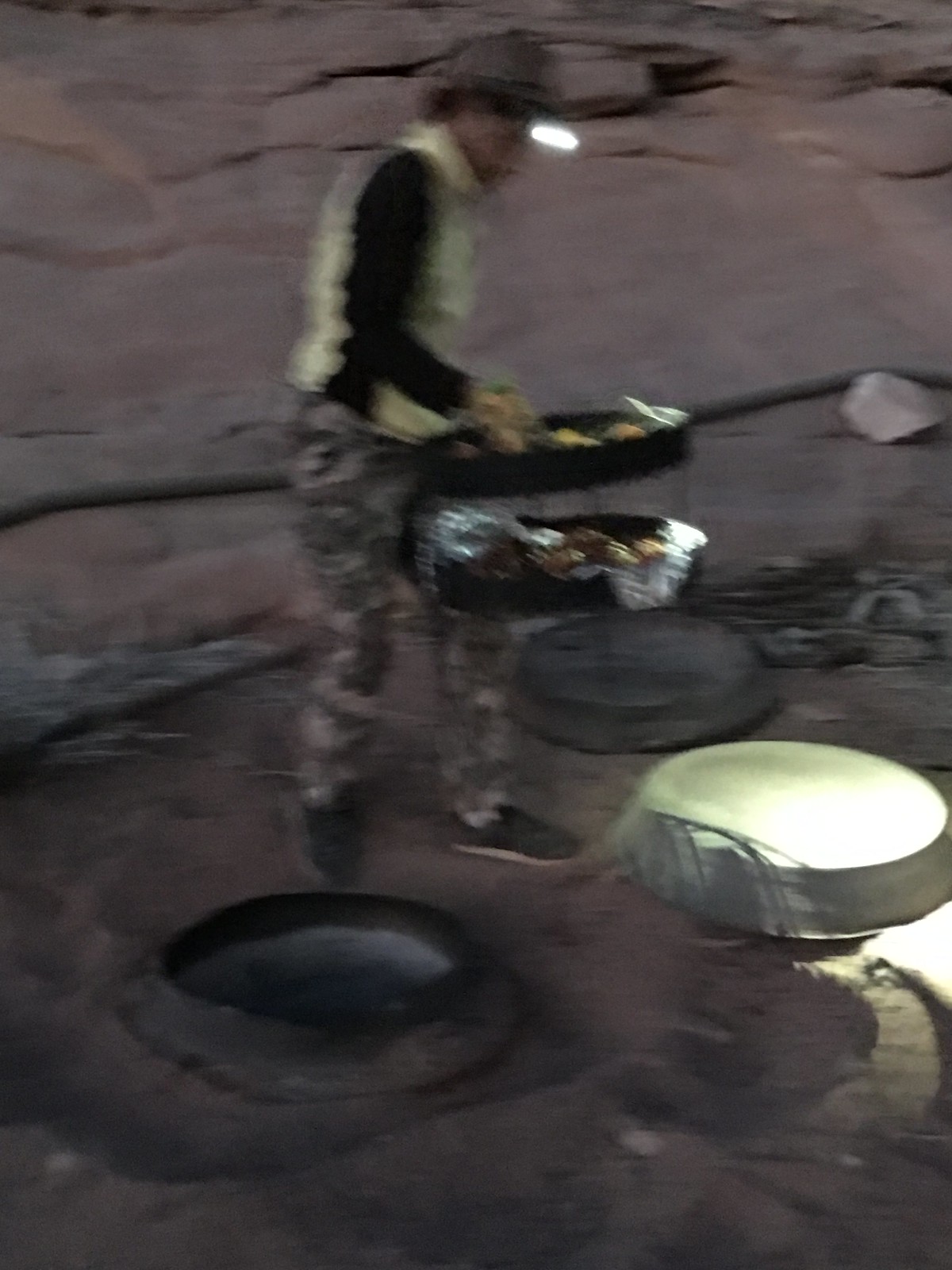The image depicts a somewhat blurry scene set against a rocky background, characterized by brownish hues dominating the top half of the picture. The bottom half features a similar rocky surface, but with a conspicuous black hole at its center. The hole appears to have had a lid, which has been removed and is now positioned towards the right side of the picture. Adjacent to the lid, there is a silver plug of comparable size. 

A single individual is visible in the scene, presumably a man, though the image's blurriness makes it difficult to discern. He is wearing a brown hat and a white vest over long black sleeves, with camouflage gray pants and black shoes that have white soles. The man seems to be holding what looks like cooking equipment, including two black pans and a piece of foil, suggesting he may be preparing for some sort of outdoor cooking activity.